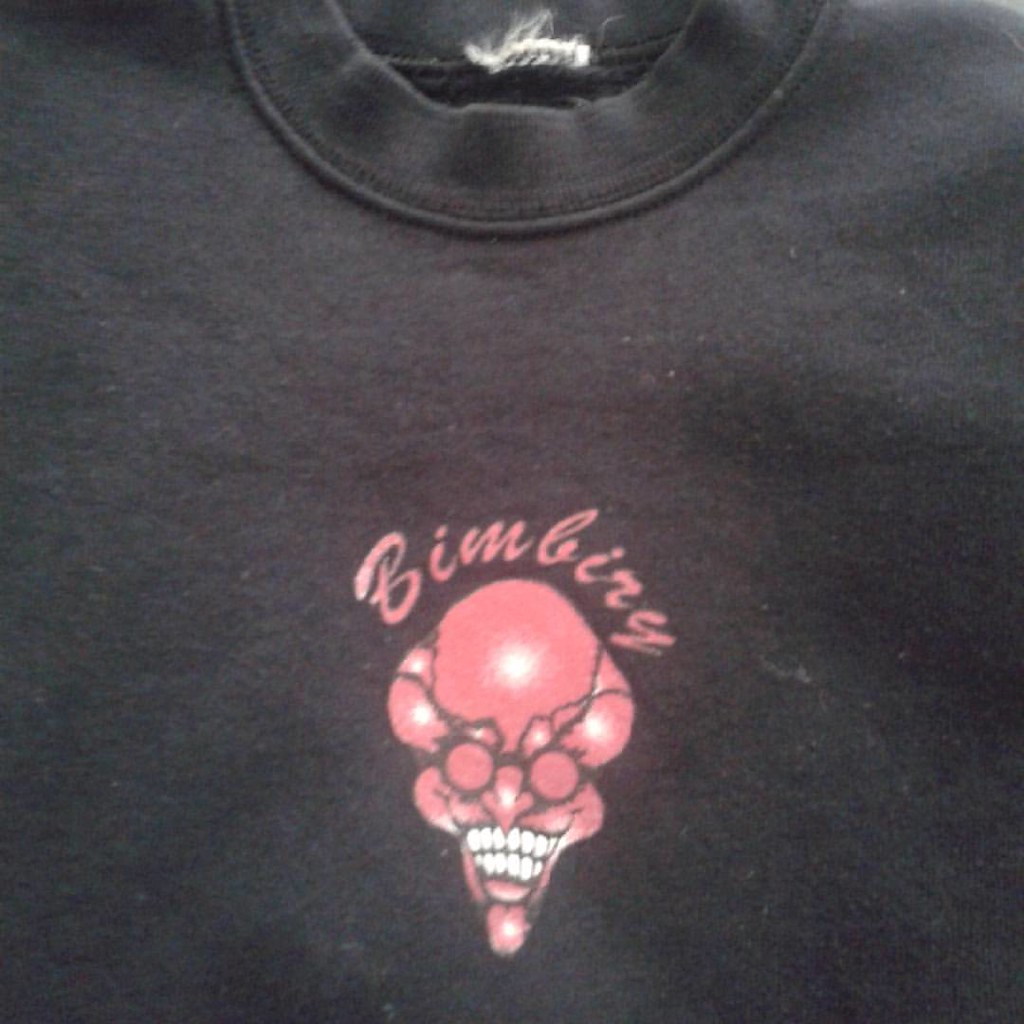A photograph captures a well-worn, black cotton t-shirt that appears somewhat faded, lending it a grayish undertone. The image quality is less than optimal, contributing to the overall vintage aesthetic of the shirt. A torn white tag is visible on the neckline, indicating its original condition. Prominently displayed on the front of the shirt is a stylized pink graphic depicting a human skull adorned with round, steampunk-inspired glasses and a noticeably narrow chin. Above the skull, cursive text spells out what appears to be "B-I-M-B-I-Z-Z" or a similar variation, though the poor image quality makes it difficult to be certain. The faded print and overall wear of the shirt suggest it might be a well-loved piece, possibly signifying a brand or logo.